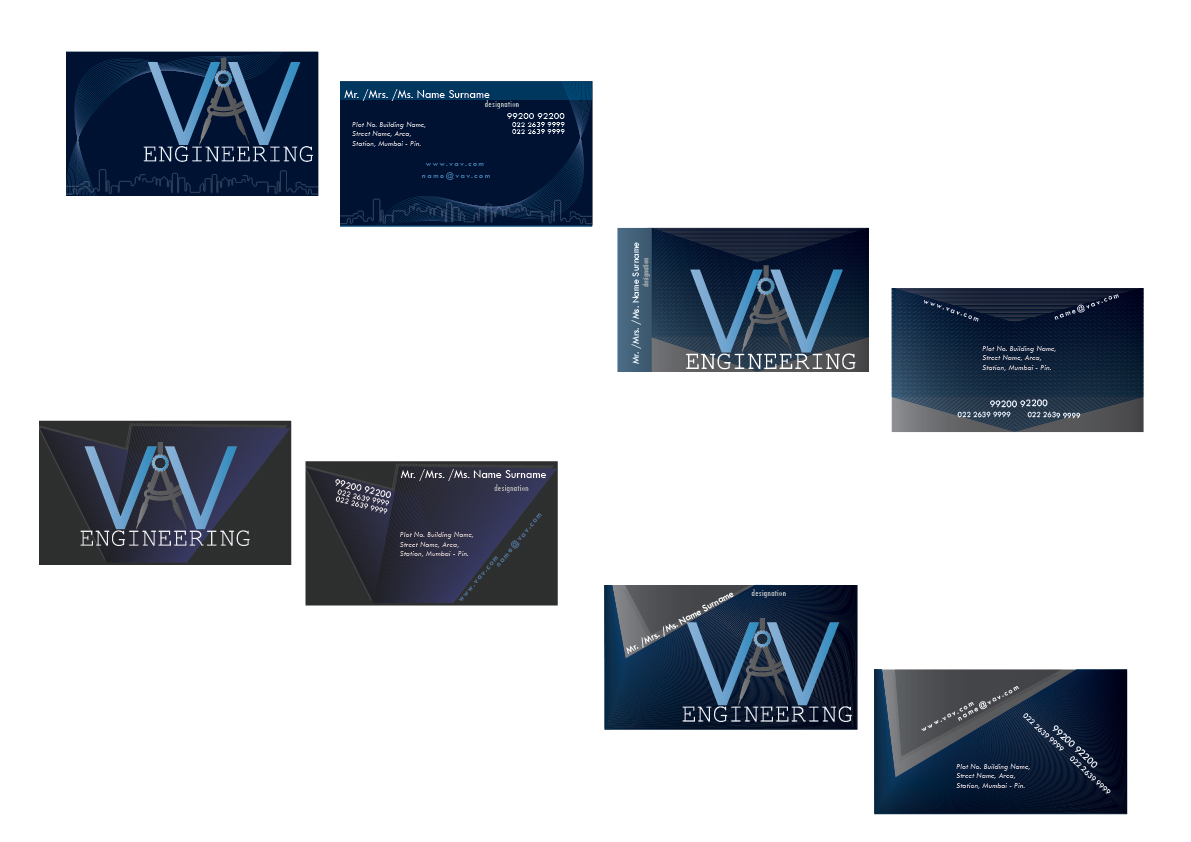This image displays a meticulously arranged series of promotional or business cards for an engineering company, likely intended for use in an advertisement or PowerPoint presentation. The cards are organized in two identical sets of four, with each set arranged in a stepped manner. The focal point of these cards is the logo "VAV Engineering," prominently featuring a pair of blue V's with a silver compass, resembling the letter 'A', nestled between them. 

The background of the cards is a dark blue shade, with the detailed company logo appearing on all fronts. The top left and third cards in each set feature a cityscape outline at the bottom of both the front and back sides, whereas the other cards showcase black and gray triangular shapes. Each card includes typical contact information, such as a placeholder for titles (Mr., Mrs., Miss), name, surname, email, telephone numbers, and the website, with text rendered in light blue and positioned strategically for legibility.

The first row of four cards includes illustrated designs with a clear logo, while the second row mirrors these designs but may also feature slightly obscured or different text content. Despite variations in background elements, the cohesive presence of the VAV Engineering logo with its distinctive compass symbol threads through the entire collection, emphasizing the brand identity.